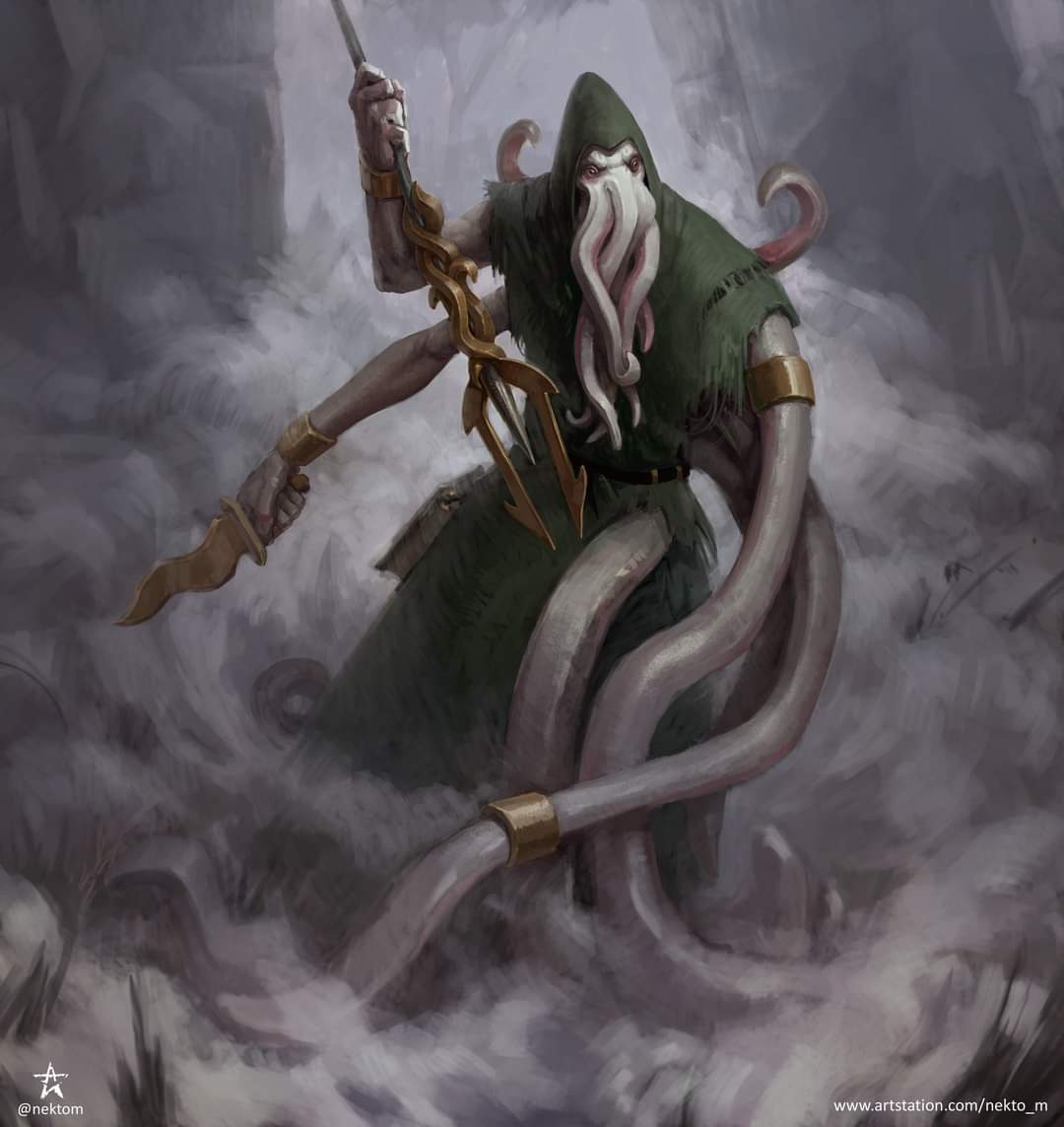This illustrated image depicts a strange, eerie creature emerging from a misty cave-like environment shrouded in smoke. The creature is a monstrous being with a hooded vest pulled up over its head, revealing two eyes and a face made entirely of writhing tentacles. It has a mix of both humanoid arms and tentacles: two arms on its left side, the upper one wielding a trident and the lower one holding a curved knife, and numerous tentacles replacing its right-side limbs, with additional tentacles protruding from its sides, hip, and shoulder blades. This creature, reminiscent of something from a comic book or video game, stands amidst swirling, smoky waves. The background, dim and indistinct, hints at a rocky, cavernous setting. In the bottom right corner, white text reads "www.artstation.com/nekto_m," while on the left side, there is a star and the username "@nektome."